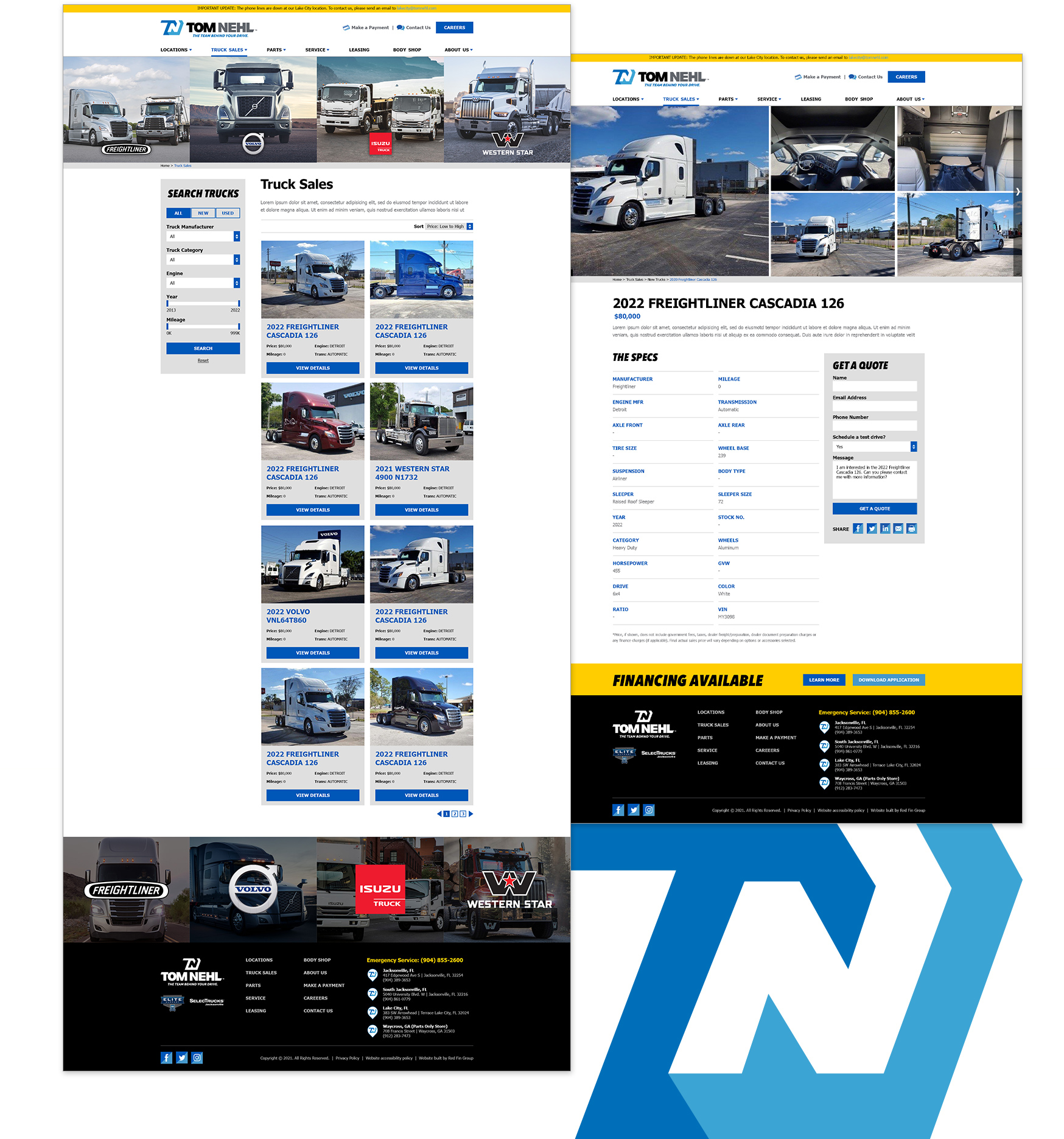This image is a composite of two webpages, presented side by side. On the left, the larger webpage features a vertical layout labeled "Tom Nell" at the top, accompanied by a company icon with the initials "T" and "N". To the right of the label, there's some text and a prominent blue button, though the content is too small to discern. Beneath this header, a photo bar showcases truck cabs, starting with a light blue truck next to a black one, followed by another light blue truck, two white trucks, and a blue truck. Below the photo bar, the section titled "Truck Sales" displays listings of trucks in two vertical columns, each featuring four trucks. The bottom of this webpage has a black bar with clickable information options like a site map.

On the right side of the composite, a specific truck from the left selection is highlighted—a 2022 Freightliner Cascadia 126. Detailed specifications of this truck are listed below the image.